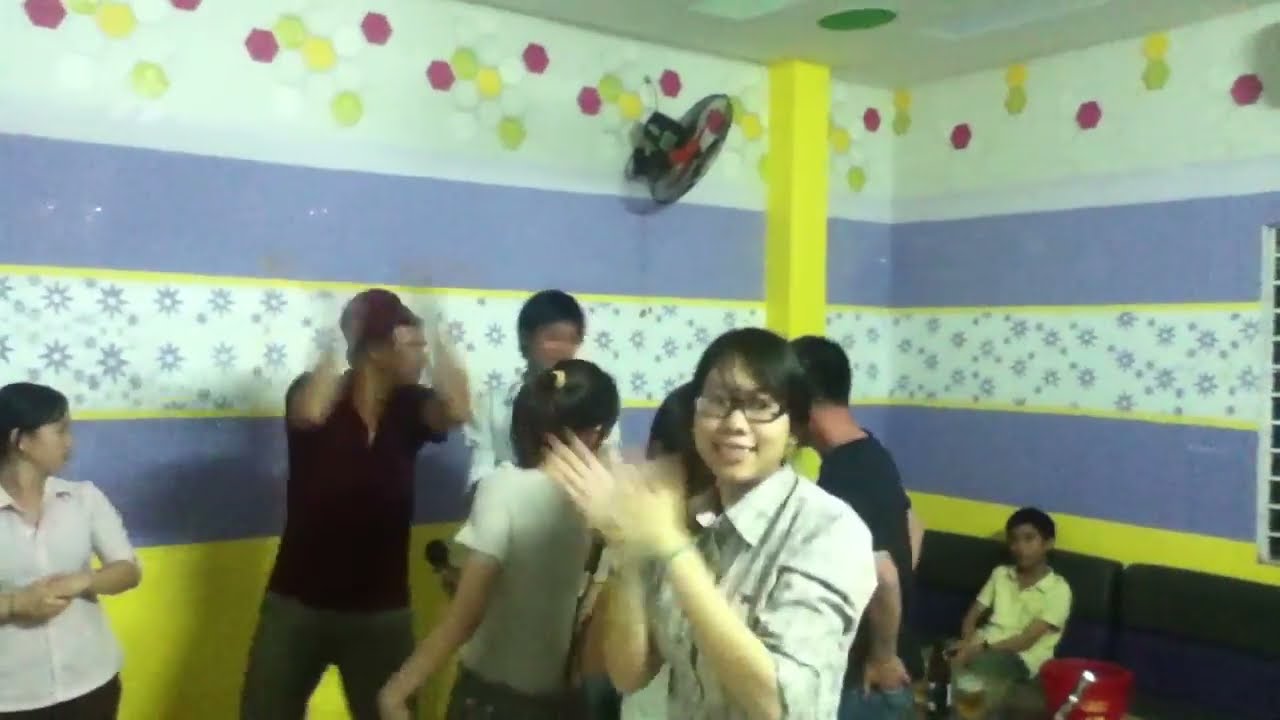In this vibrant and colorful room, which resembles a children's play area, about seven or eight people have gathered, most of them standing. The walls are adorned with a lively mix of horizontal stripes in white, blue, and yellow, embellished with designs, including purple bands, stars, and speckled spots in green, yellow, and pink. A black fan is mounted high on one of the walls. A few people, including a woman with glasses wearing a khaki shirt, are captured mid-clap, their hands a blur, indicating an atmosphere of celebration or a party. In the foreground, the clapping woman stands prominently, while in one corner of the room, a young boy in a yellow shirt sits on a black and purple sofa, next to a table laden with bottles and a red bucket. This colorful and lively scene appears to feature mostly Asian people enjoying a festive moment together.